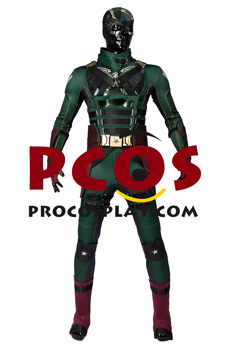The image depicts an action figurine resembling a humanoid character from a video game. The background is plain white, making the figure stand out prominently. The figurine is garbed in a predominantly green and black suit, featuring metallic elements. It sports a shiny black face mask with metallic green hair. The green, long-sleeved shirt has a large neckline reaching almost to the chin, complemented by a black vest embroidered with green horizontal lines and touches of gold, and sections with silver accents. The figure has black bands across its chest and dark green tights, under which black shorts are visible. The figurine also wears dark red boots with black tips. Its hands are positioned downward by its sides. Striking red letters across the top spell out "PCOS," with a yellow highlight beneath the letter 'O' and an additional smaller, less legible text underneath.